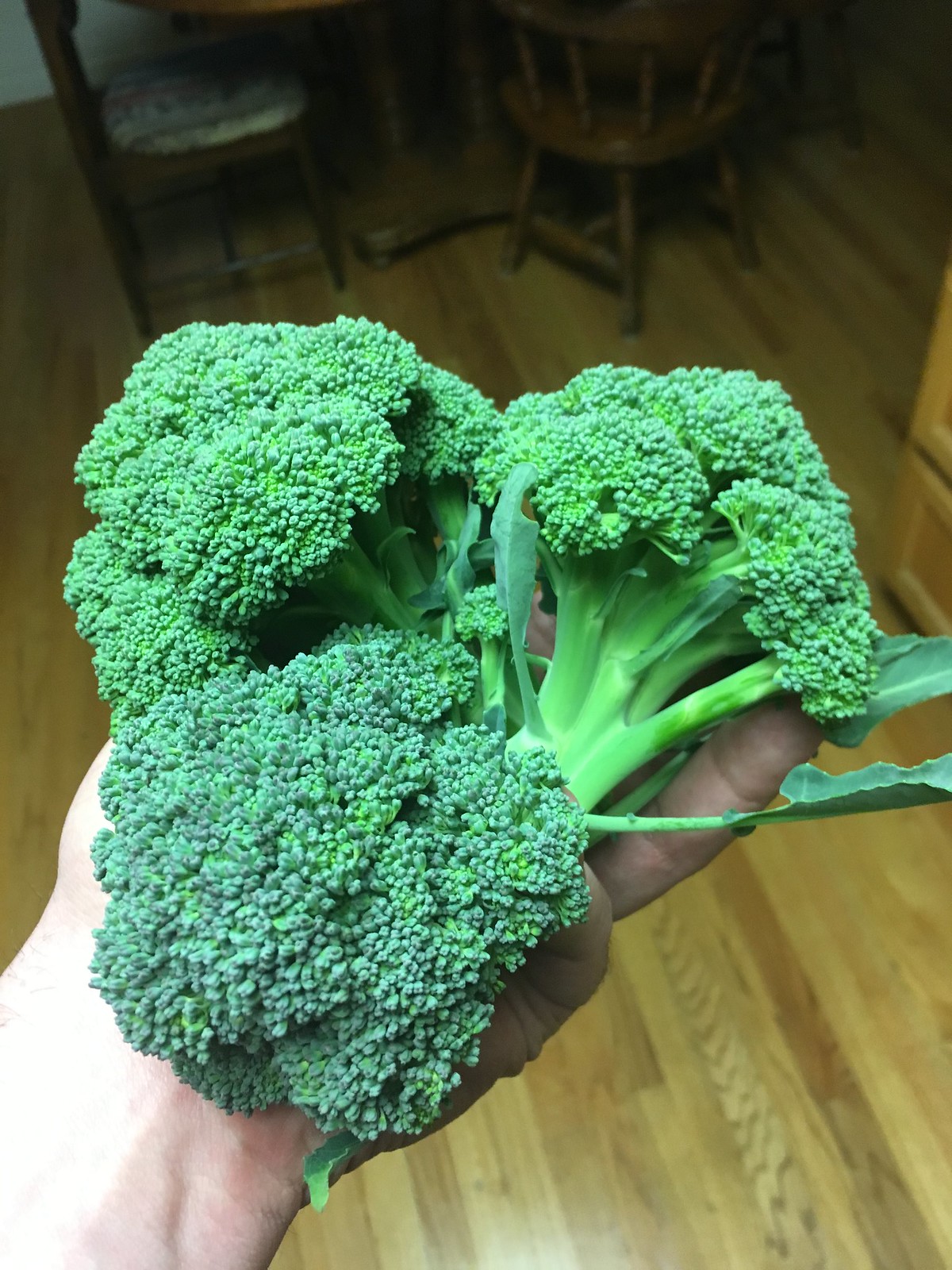This overhead photograph captures a detailed scene within a dimly lit dining or kitchen space, featuring an intriguing composition centered around a hand holding three large, tree-shaped broccoli heads. The hand, likely belonging to a white male, is prominently displayed in the foreground, with the vibrant, green broccoli crowns, complete with attached leafy sections, almost entirely covering his palm. The background reveals a wooden slat floor, characterized by narrow strips of wood, and faint glimpses of wooden furniture, including a dining table with visible table legs and two chairs—one of which has a white cushion. Additional elements, such as the edge of a countertop or cabinet, subtly intrude into the scene, adding depth to the indoor setting. No text accompanies this rich and vibrant image, which starkly contrasts the bright, fresh green of the broccoli with the muted tones of the room.